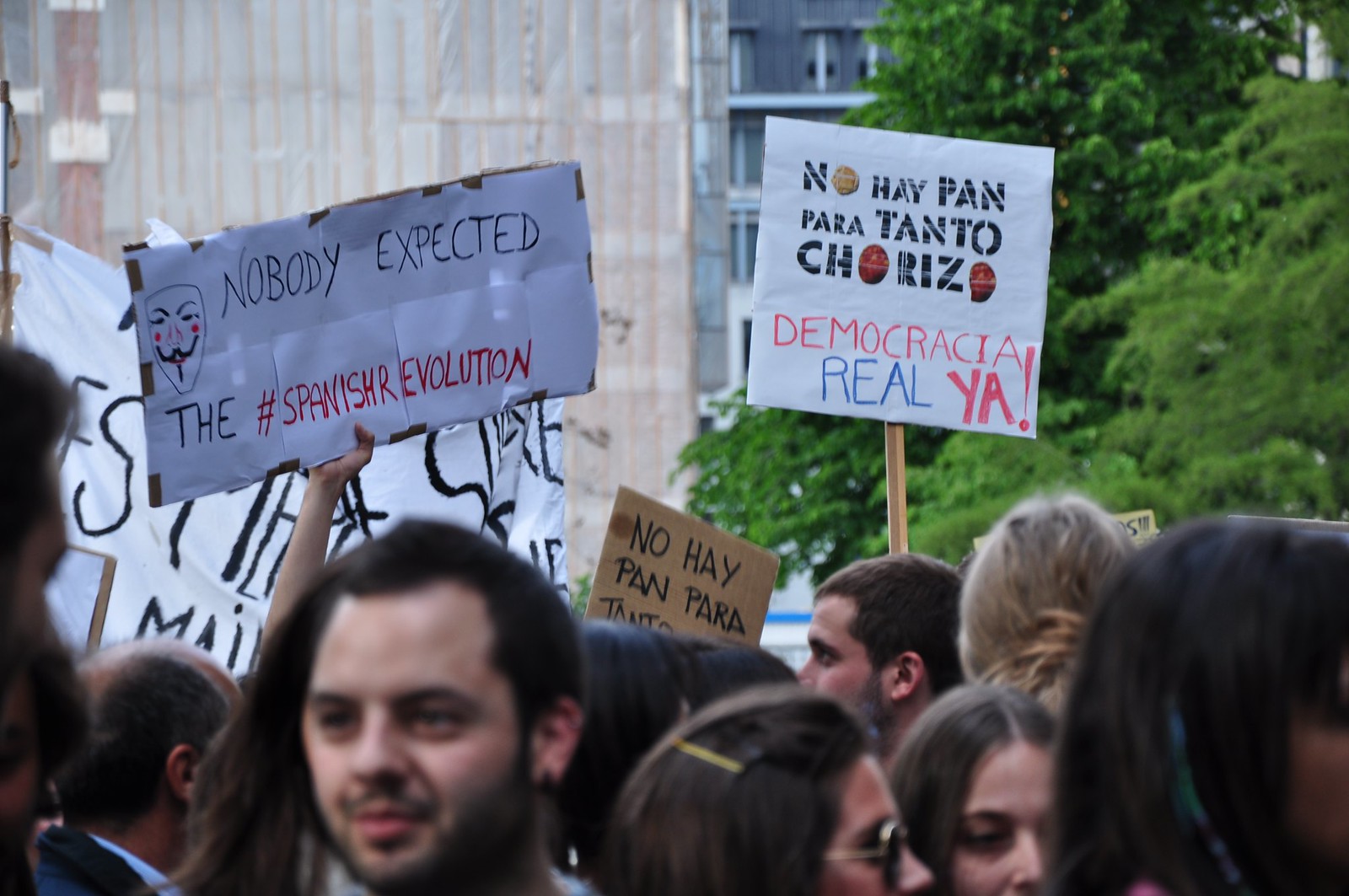This color photograph captures an urban street protest with a group of people holding signs, indicating their participation in a demonstration. The backdrop features a gray building with windows and a few trees, suggesting the location might be near a park or an urban area with greenery. Among the protestors, many of whom have lighter skin tones, the signs are primarily in Spanish. One prominent sign displays imagery from the movie "V for Vendetta" and reads, "Nobody Expected the #SpanishRevolution."

Notably, a sign reads, "No Je Pan Para Tanto Chorizo Democracia Real Ya," while another cardboard sign partially reads, "No Je Pan Para." In the foreground, a man with dark, short hair, an earring, mustache, and beard faces the camera directly. Beside him, a woman with dark hair and sunglasses faces away, and a blonde girl can also be seen with her back to the camera. The detailed expressions and varied directions of focus among the protesters add depth to the scene's dynamic atmosphere.